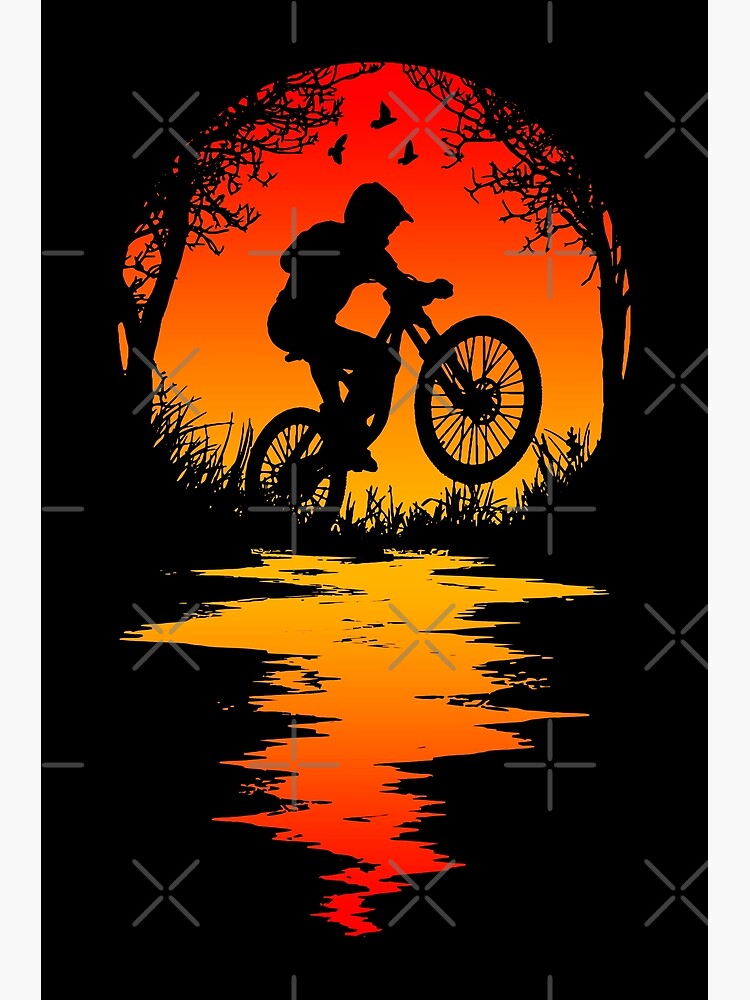The digital artwork depicts a dramatic silhouette of a man performing a wheelie on a dirt bike, surrounded by a night sky teeming with visual elements. Captured from a low vantage point that appears to be inside a sewer, the scene shows the rider emerging and accelerating away. Dominated by hues of black and orange, the image features a setting sun whose vibrant, fiery reflection illuminates the water surface below. The sky hosts three black silhouette birds flying near the top, adding to the dynamic composition. Leafless trees with stark branches frame the rider on both sides, their dark forms contrasting sharply against the bright gradient of the sunset. Scattered throughout the poster are various crosses and plus marks, contributing to its intricate design. The overall impact is a visually-stunning depiction of motion and stillness, all rendered in striking monochromatic tones except for the illuminating sun and its reflections.